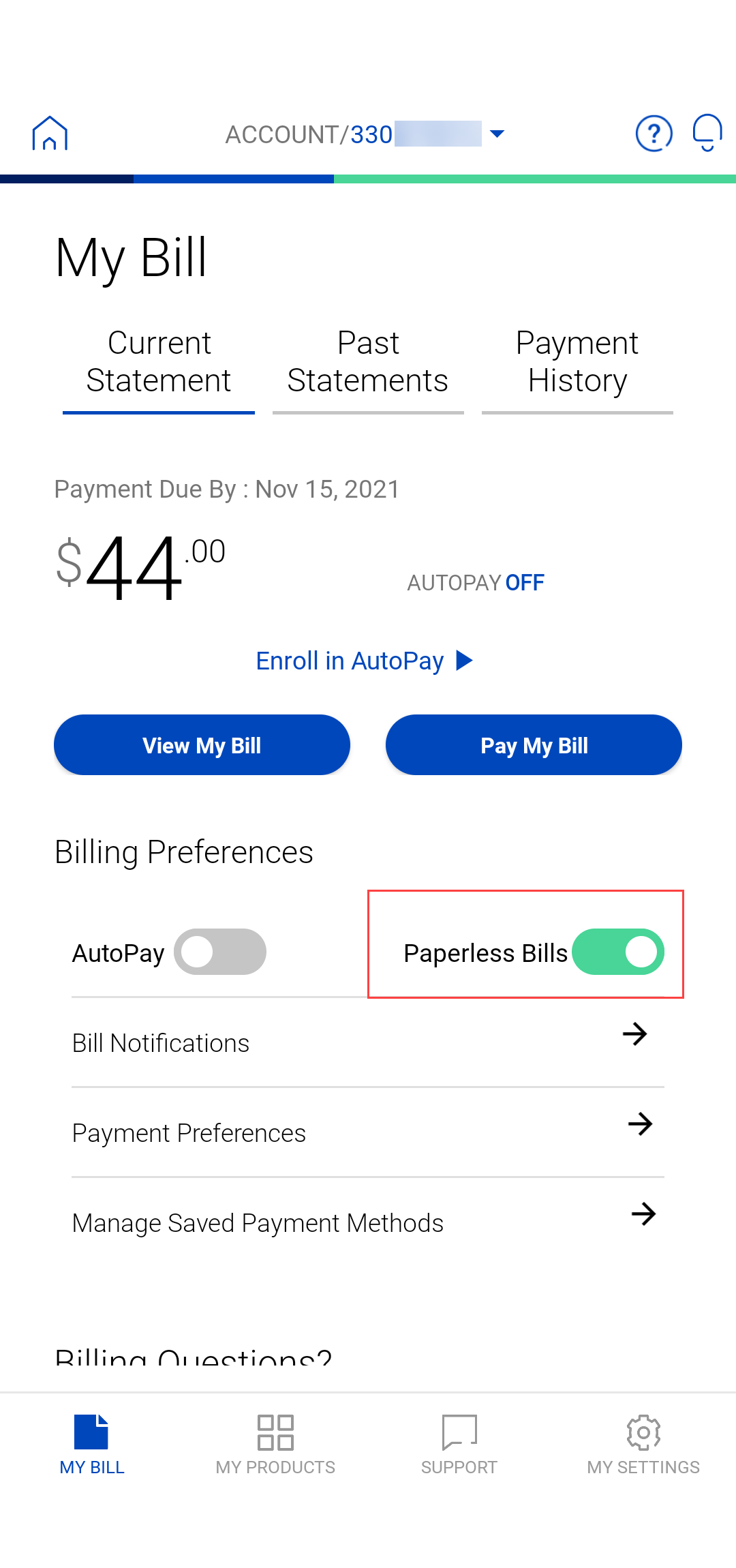The image displays the "My Bill" page of an account interface. At the top left corner, there's a "Home" button. Centered on the same line is the text "Account / 330," with the rest of the account number redacted, followed by a drop-down arrow. To the right, there is a circular icon with a question mark inside, and a bell icon for notifications. Below this toolbar is a horizontal separator bar.

In the main content area, a section labeled "My Bill" appears on the left. Directly below this heading, there are three tabs: "Current Statement," "Past Statements," and "Payment History," arranged side by side. The "Current Statement" tab is selected. 

Under "Current Statement," it indicates "Payment Due by November 15, 2021," with the amount listed as $44 beneath it. To the right of the due amount, it displays "Auto Pay Off." Centered below this information is an option labeled "Enroll in Auto Pay." At the bottom of the section, there are two buttons: "View My Bill" and "Pay My Bill."